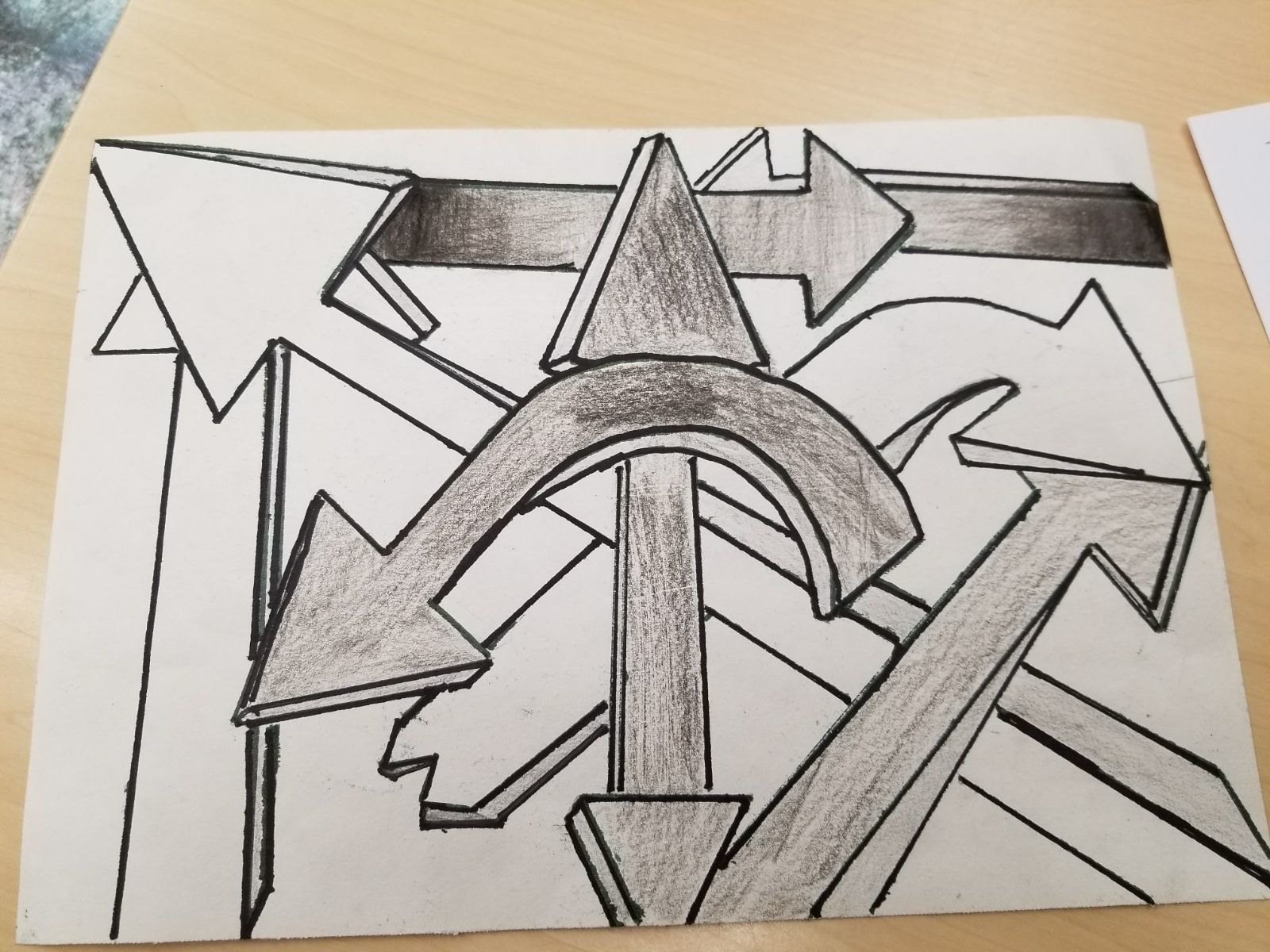The image features a detailed pencil or crayon drawing on a sheet of paper, which is situated on a light pine wood table with a polished finish. To the right side of the primary drawing sheet, there is the corner of another piece of paper. Additionally, in the top left corner of the image, a small segment of light blue carpet or fabric is visible off the edge of the desk.

The drawing itself includes multiple arrows. In the bottom left corner, there is a curved arrow that arcs downward. Adjacent to this arrow, there is a vertical up-down arrow. Further to the bottom left of these, an upright arrow is positioned, and all three of these arrows are filled in with black shading. Overlaying these, there is a large arrow that extends from the bottom right corner towards the top left corner, remaining unshaded and colored white. Underneath the head of this large white arrow, another arrow points straight upwards from the bottom of the page.